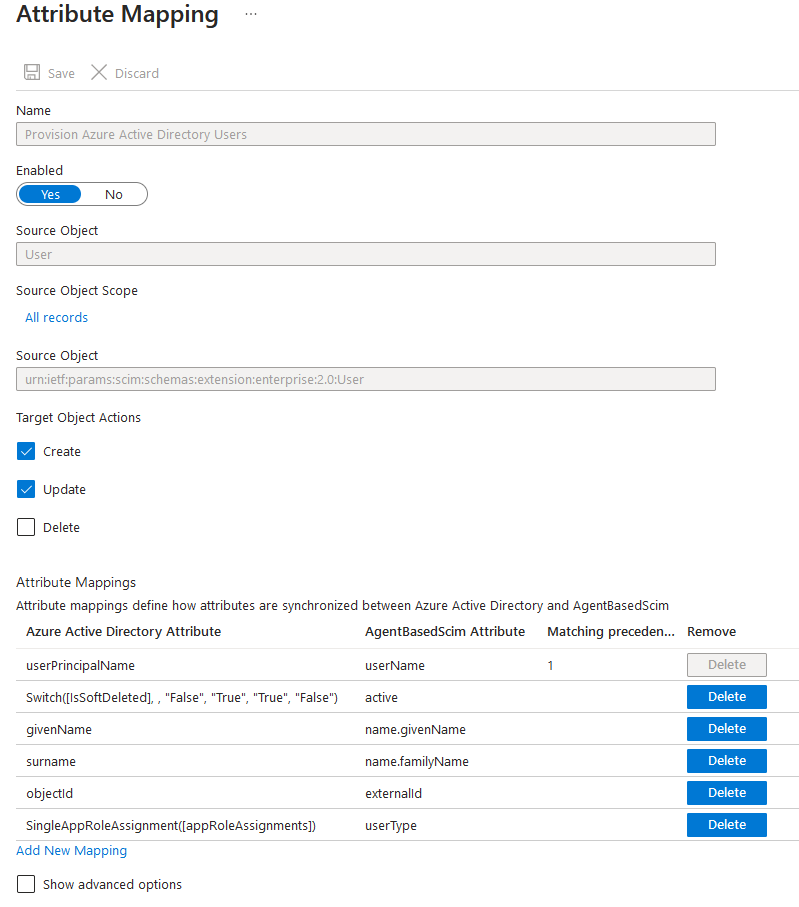The image displays an interface on a white background featuring black text. At the top, the title "Attribute Mapping" is prominently displayed. Two buttons labeled "Save" and "Discard" are situated below the title, offering options to either save the changes or discard them.

Below these buttons, there is a gray text box labeled "Name" with the input "Provision Azure Active Directory users." Adjacent to this is the label "Enabled," accompanied by a toggle switch set to "Yes."

Further down, the interface presents several labeled text boxes and options:

- **Source Object**: "User"
- **Source Object Scope**: "All Records"
- **Source Object**: (specific address point provided)
- **Target Object Actions**:
  - "Create" (checkbox checked)
  - "Update" (checkbox checked)
  - "Delete" (checkbox not checked)

Subsequently, additional details about attribute mappings are provided:

- **Attribute Mapping**: A note indicates that attribute mapping defines the synchronization between Azure Active Directory and agent-based DSCIM.
- **Azure Active Directory Attribute**: "User Principal Name" synchronized with "Username"
- **Switch**: 
  - "False" 
  - "True"
  - "True"
  - "False"
  - "Active"
- Mapping details include:
  - Given Name: "name.givenName"
  - Surname: "name.familyname"
  - Object ID: "externalId"
  - Single App Role Assignment: "appRoleAssignments"

An option to add a new mapping is available, along with a checkbox labeled "Show advanced options," which is currently unchecked.

The detailed description ensures that each element and option within the interface is clearly and comprehensively described.